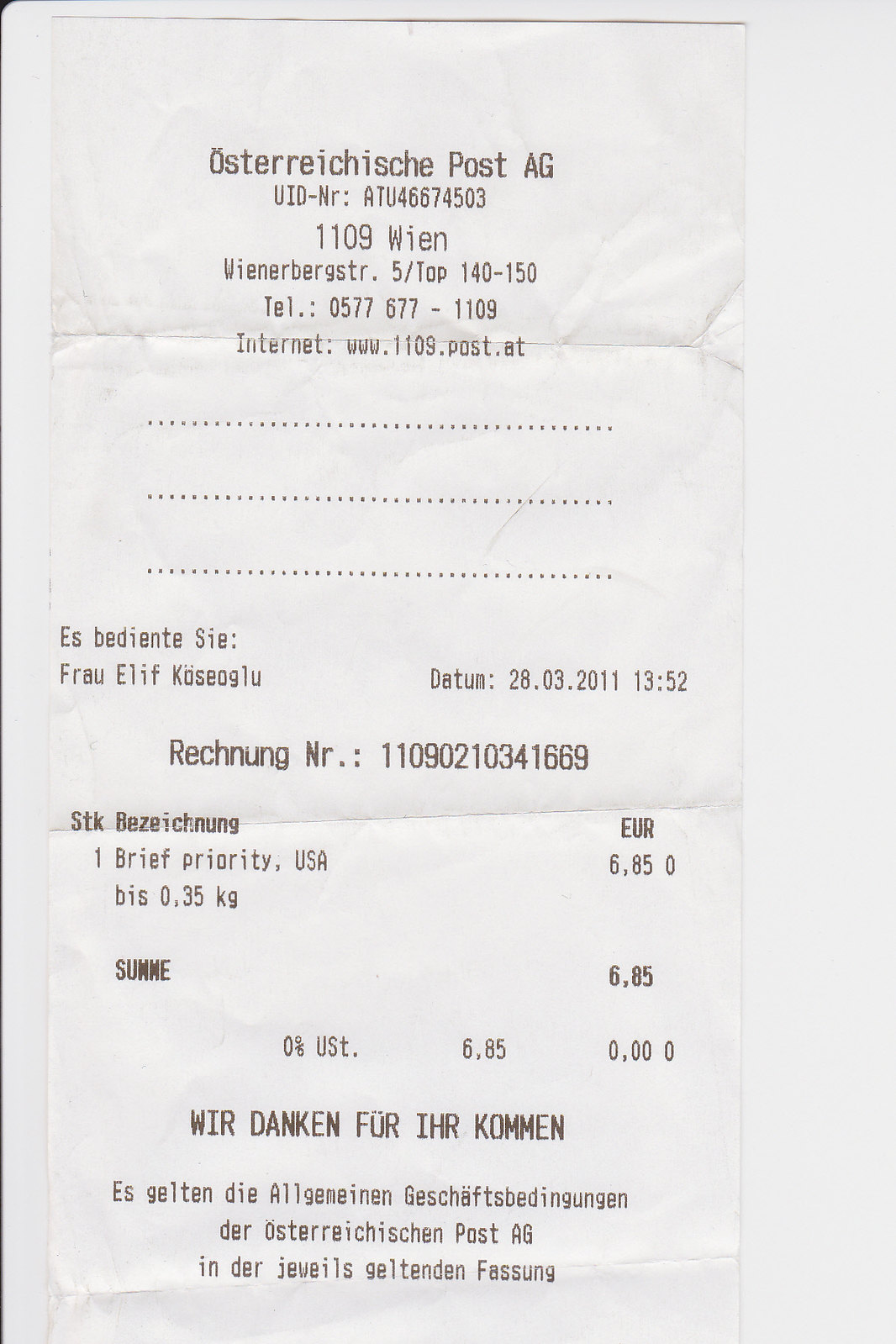The image shows a detailed paper receipt from the Austrian store Osterreichische Post AG, located at 1109 Vienna (Wien). The receipt, set against a light gray background, is printed in black ink on traditional white paper. At the top, the receipt header includes the store's name and its identification details such as UIDNR and the location number 1109WIEN. It also provides the website www.1109.post.at. Midway down the receipt, three horizontal dotted lines separate the header from the body of the receipt. Below these lines, the itemized section details the transaction: sending a priority package (Brief Priority USA) to the United States costing 6.85 Euros. The receipt includes a total price of 6.85 Euros. Text at the bottom reads, "Wir danken für Ihr Kommen, es gelten die allgemeinen Geschäftsbedingungen der Österreichischen Post AG in der jeweils geltenden Fassung," indicating gratitude for the visit and referring to the store's general terms and conditions.